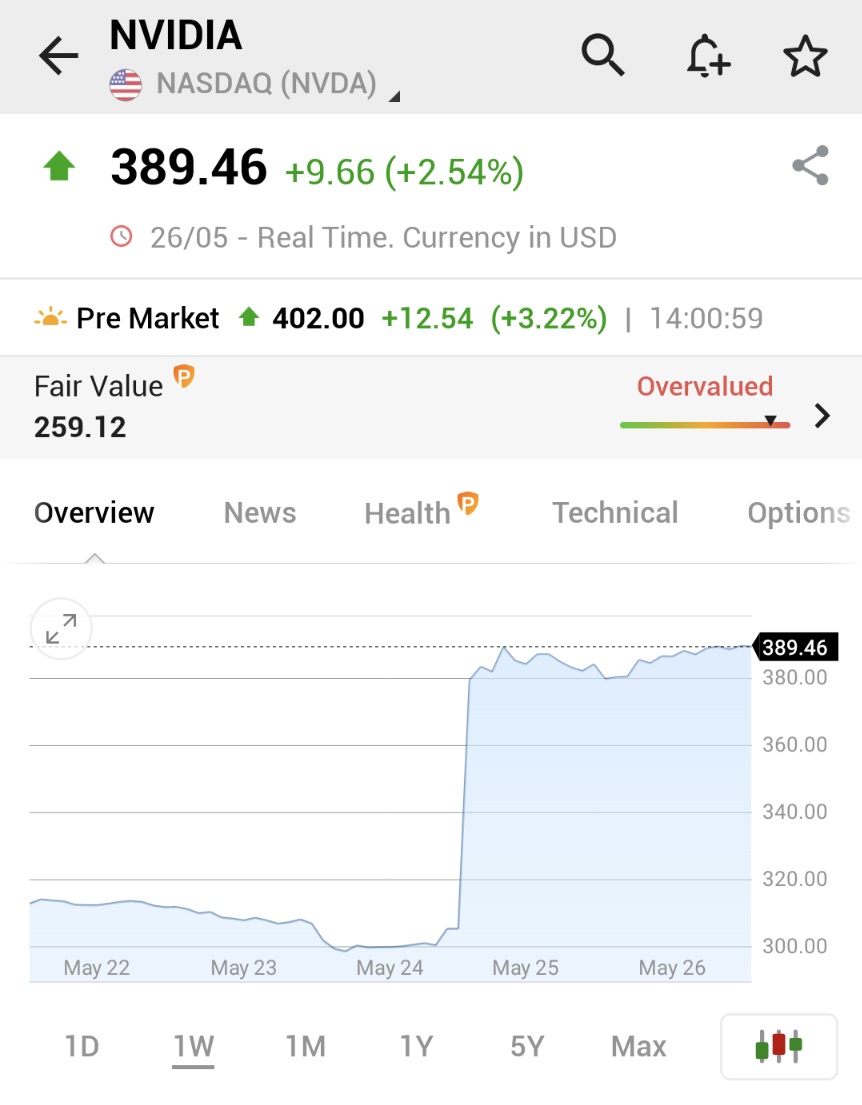This screenshot captures comprehensive stock information for NVIDIA, as displayed on a financial analysis platform.

At the top of the interface, the header contains a prominent gray box with a back arrow on the left. The name "NVIDIA" is centrally displayed, accompanied by a circular icon featuring an American flag, indicating the stock is traded on NASDAQ (NVIDIA). Adjacent to this text are three icons: a search icon, a bell (notification) icon, and a star (favorite) icon, lined up from left to right.

In the next section, the current stock price is highlighted. "389.46" is shown with a green arrow pointing upwards, indicating an increase. This change is further detailed as "+9.66," which equates to a "+2.54%" rise. Information about real-time data and the currency being in USD is also present in this section.

Below that, there is a pre-market data segment featuring a half sun icon. Here, another green arrow points upward next to "402," showing a pre-market increase of "+12.54," equivalent to "+3.22%." The time of this data is also included.

The section that follows is labeled "Fair Value," which lists "259.12." To the right of this value, red text states "Overvalued," complemented by a temperature-like bar that transitions from green to red, visually depicting the stock's valuation status.

The interface also features a row of categories: Overview, News, Health, Technical, and Options, providing different perspectives and detailed insights into the stock's performance.

Below these categories lies a graphical representation of NVIDIA's stock performance. The graph includes a Y-axis with prices and an X-axis with dates, enhancing the temporal context. Additional options allow the user to view data across different timeframes: one day, one week, one month, one year, five years, and a maximum range. A settings button is situated to the right of these options, presumably allowing further customization of the display.

Overall, the screenshot offers a thorough snapshot of NVIDIA’s stock performance, valuation, and market behavior in an organized and user-friendly manner.